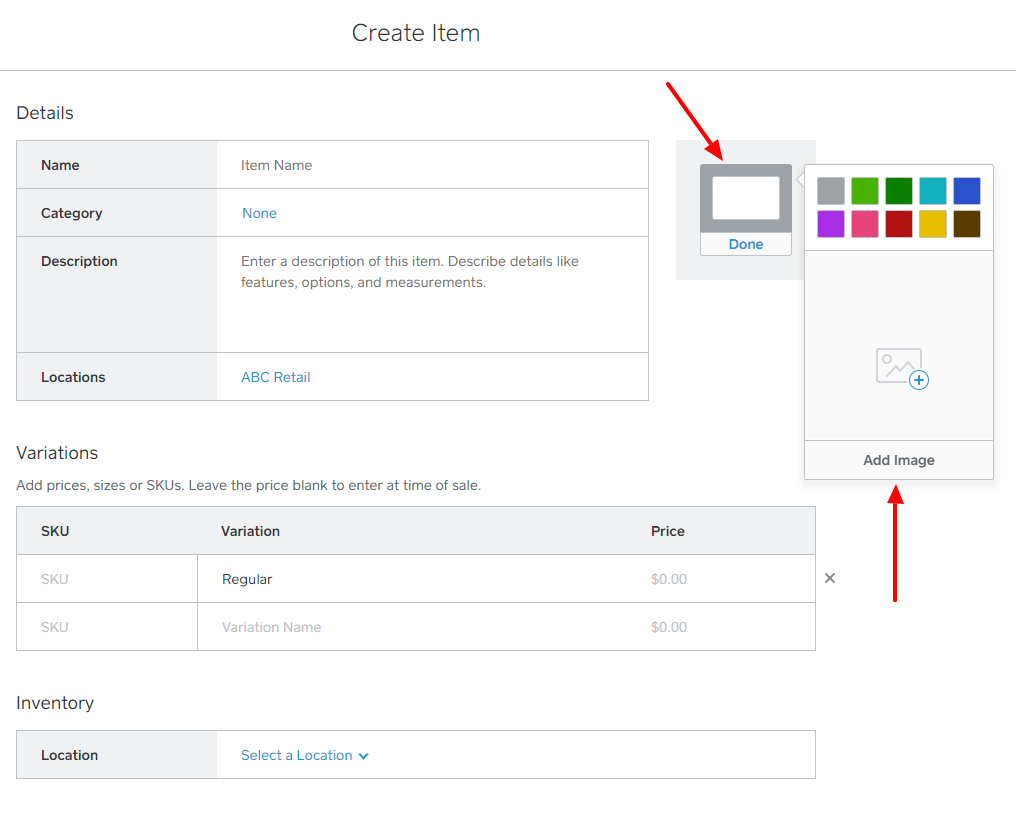The interface displays a section titled "Create Item" at the top with a light gray horizontal line beneath it. Below this line, the word "Details" is prominently featured. On the left side, there is a gray column, while on the right side, there is a white column. The grey column lists fields vertically: "Name," "Category," "Description," and "Location." Correspondingly, the white column contains:

1. Under "Name," it says "Item Name."
2. Under "Category," it says "None."
3. Next to "Description," it has the prompt "Enter a description of this item, describe details like features, options, and measurements."
4. Under "Location," it says "ABC Retail."

To the right, there is an image of a box with the word "Done" beneath it, indicated by a red arrow. Adjacent to this, there is another box labeled "Add Image" at the bottom, also highlighted by a red arrow. Additionally, atop this second box, there are ten squares in various colors: gray, light green, dark green, light blue, dark blue, purple, magenta, brown, and black, with a photo icon positioned underneath them.